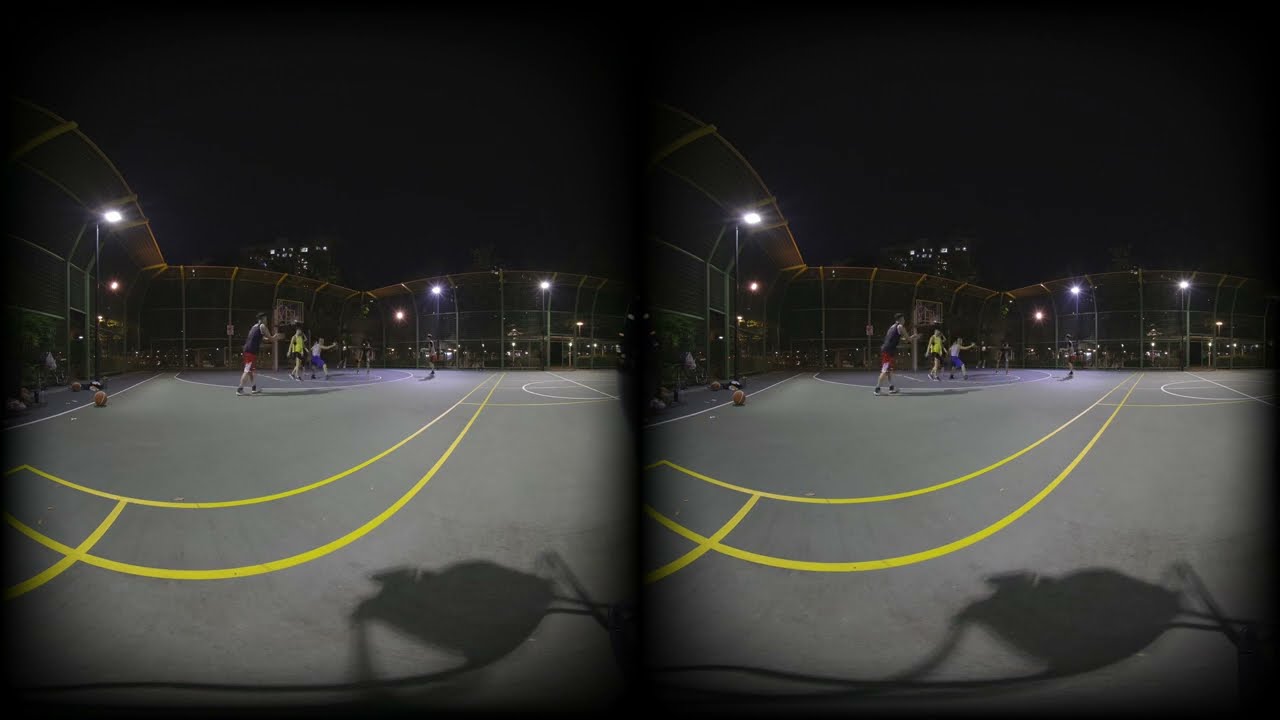In this image, there are two identical pictures side by side, each depicting an outdoor nighttime basketball game. The court, lit by about six bright light posts, features gray concrete with yellow and white markings, including a prominent yellow three-point line that curves around the playing area. A building in the background is illuminated, providing additional context to the urban setting. 

On the court are four visible players: one in a black tank top with red shorts, another in a yellow tank top with gray shorts, a third player wearing a light blue shirt, and a fourth in a gray shirt with red shorts. The player in the black tank top appears to be preparing to shoot a three-pointer. Additional figures can be seen waiting on the sidelines, suggesting others are ready to join the game. 

The top, bottom, and sides of the image are blacked out, giving a sense of viewing through goggles, which has resulted in a curved, distorted effect at the front of the picture. The scene is framed by a silver gate, with a dark, city skyline silhouetted in the background. An orange basketball is visible on the court, and shadows can be seen in the right-hand corner, adding to the dynamic feel of the image. The overall symmetry and repetition of the identical images create a unique visual effect, emphasizing the urban basketball ambiance at night.